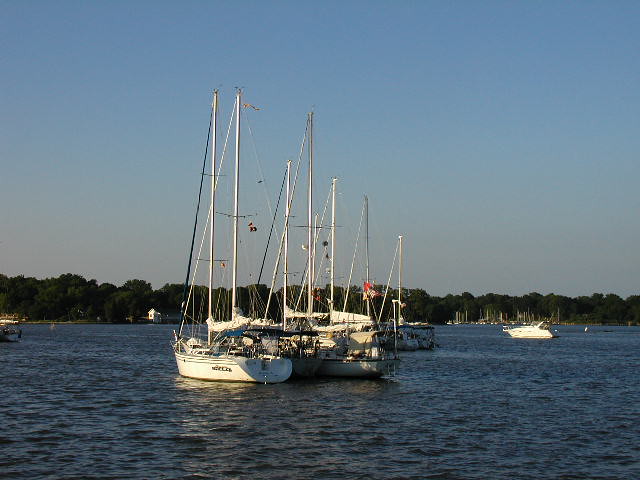This vibrant outdoor photograph captures a serene lakeside scene under a bright blue, cloudless sky. Dominating the midsection of the image are three white sailboats clustered together in a calm, dark blue lake. These boats, appearing like yachts with large, bare masts, reflect sunlight from the left, hinting at a sunny day despite the absence of visible clouds. To the right of the sailboats, a white pontoon boat cuts across the water, heading left. The distant horizon reveals a dense tree line stretching across the shore, with a small white patch breaking the continuity, perhaps a gap in the foliage. The farther background features numerous indistinct boats, mostly sailboats, dotting the watery expanse, adding to the tranquil ambiance of the scene.